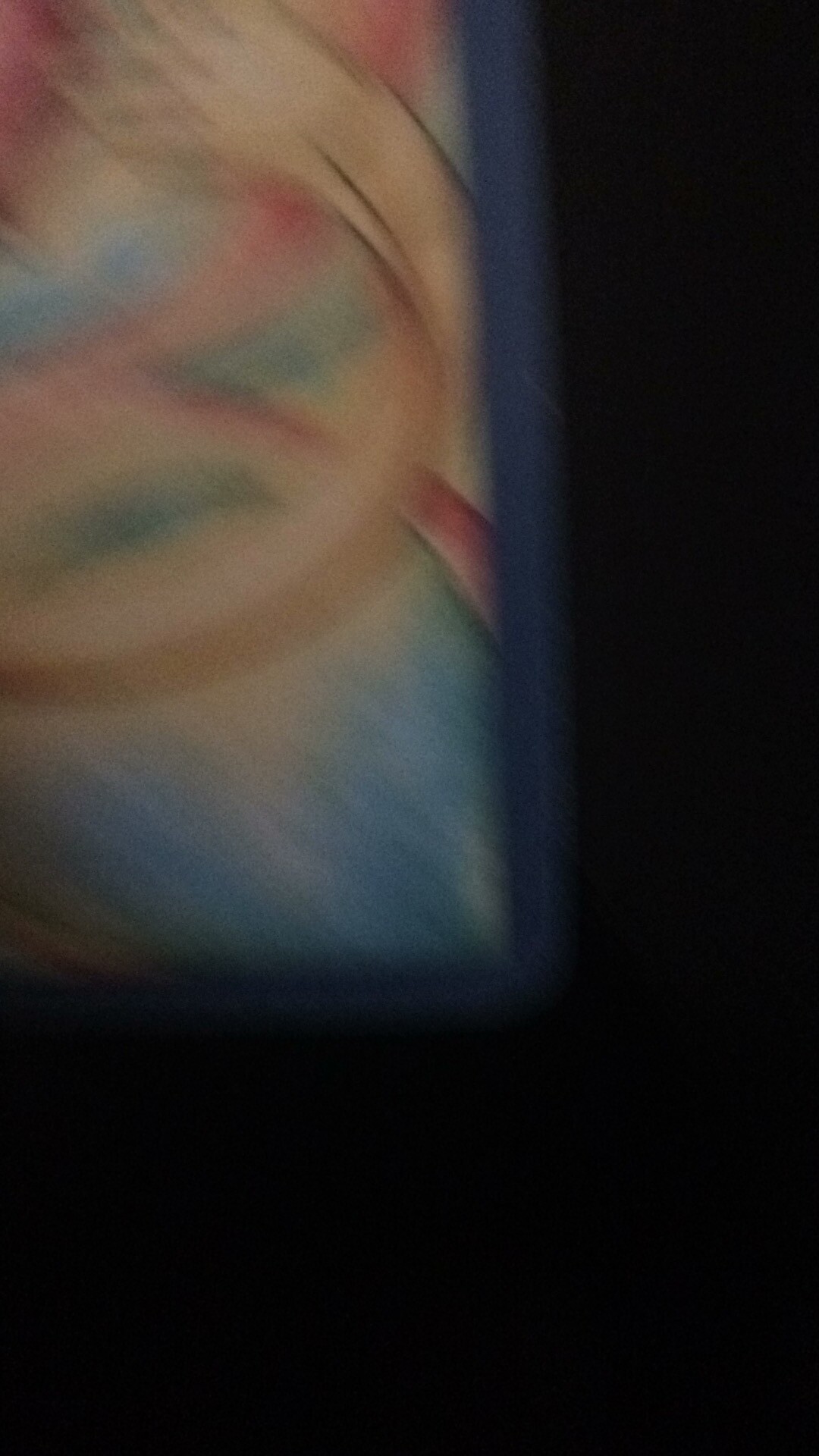The image appears to be an out-of-focus photograph with a predominantly black background forming an L-shape along the right side, bottom, and part of the left side. The image is framed by a dark blue border that lightens into a cream color at the bottom. Within this frame, there are abstract, blurry shapes in various colors, including red, green, brown, white, and black outlines. An orange half-circle reaches from the left side, fading as it moves inward, and there is another orange or red strip on the right side, which similarly fades towards the center. Above this strip, an orange crescent extends with what resemble fingers or ends, accented by white, brown, and some blue and green hues. The vague impression of a distressed cartoon character is also suggested, with elements such as a blue shirt, blonde hair, a downturned blue mouth, and blue-shaded eyes being mentioned, though these features are indistinct due to the blurriness. The overall effect is reminiscent of a stained-glass window or a drawing with a colorful yet unclear composition.